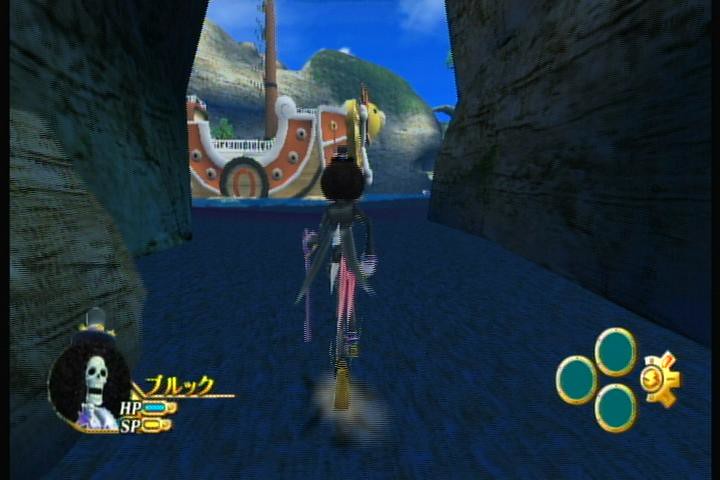The image appears to be taken from a video game, showcasing an intricate and immersive setting. The bottom of the screen features a blue surface that resembles a carpet, poised within a towering tunnel that stretches skyward. In the center of the scene, there's a body of water accompanied by a red, u-shaped ship adorned with gold dots, as well as a vertical pole ascending upwards.

On the right side of the screen, there are three green circles and a semi-circle that resembles a yellow half-sun. To the lower left, a black circle displays a skeleton head along with HP (Health Points) and SP (Stamina Points) bars. The player's character stands out with very skinny pink legs and a slender black body, topped off with what looks like a black circular beret viewed from behind, adding a unique flair to their appearance. The character design suggests that the player may actually represent the skeleton shown in the lower left interface.